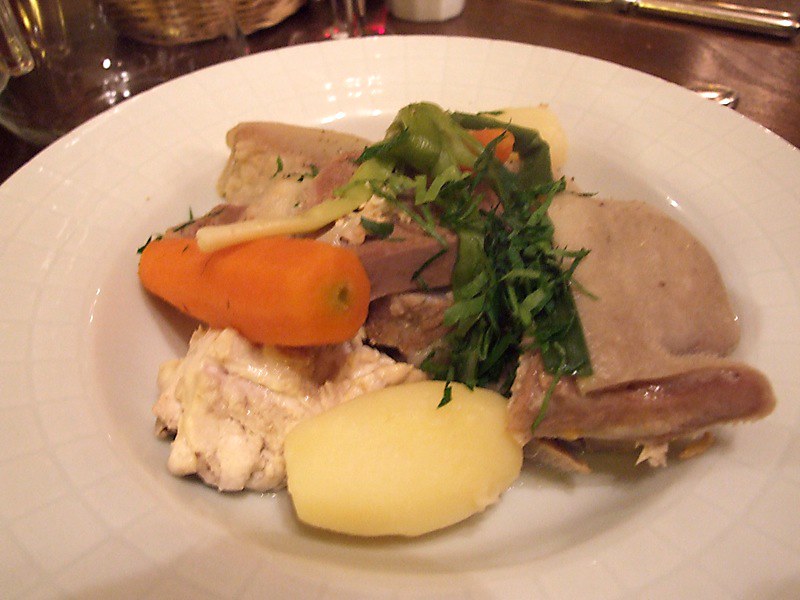The image captures a detailed, though somewhat unappetizing, presentation of food on a white porcelain dish with a subtle concave design and embossed rectangle pattern around the edge. The dish contains a mix of steamed and mashed potatoes, a roasted carrot, sliced pork, sauerkraut, and a few green leafy herbs, possibly cilantro or boiled green onions. The food is arranged haphazardly. The plate is set on a wooden table, suggesting an indoor setting likely in a restaurant or dining room. In the background, you can see a couple of pieces of silverware with indistinct handles and a partially visible clear glass or jug, along with the very bottom of a white wicker basket. The image quality is grainy, adding a layer of ambiguity to some details.